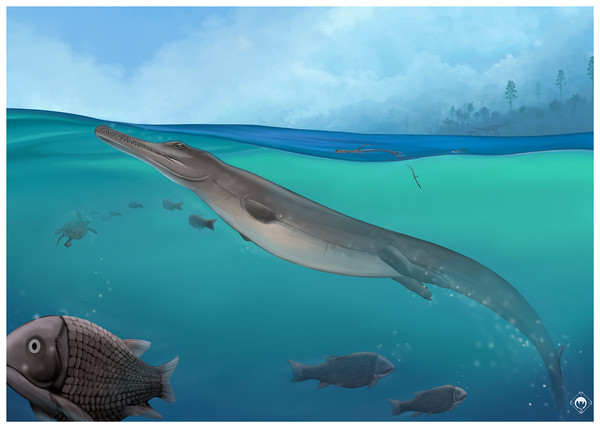The image is a detailed landscape-oriented illustration portraying a prehistoric aquatic scene. Dominating the center is an ancient creature that resembles a crocodile but with distinct features that blend characteristics of both a fish and a caiman. Its body, colored in a grayish hue reminiscent of a shark, stretches from its head positioned towards the left to its tail tapering to the right and slightly downward. This creature has stubs instead of fully-formed legs, and its wide, flat snout is lined with sharp teeth.

Immersed in a cross-sectional view of water, the scene showcases a variety of aquatic life. Several fish are scattered throughout, with a noticeable presence near the bottom left of the image. A turtle can also be seen swimming on the left side. 

Above the water, the sky is depicted as mostly cloudy with patches of blue peeking through. In the top right background, faint silhouettes of trees, bushes, and what appears to be a brontosaurus add depth and context to the prehistoric setting. A small white logo is visibly placed in the bottom right corner of the artwork.